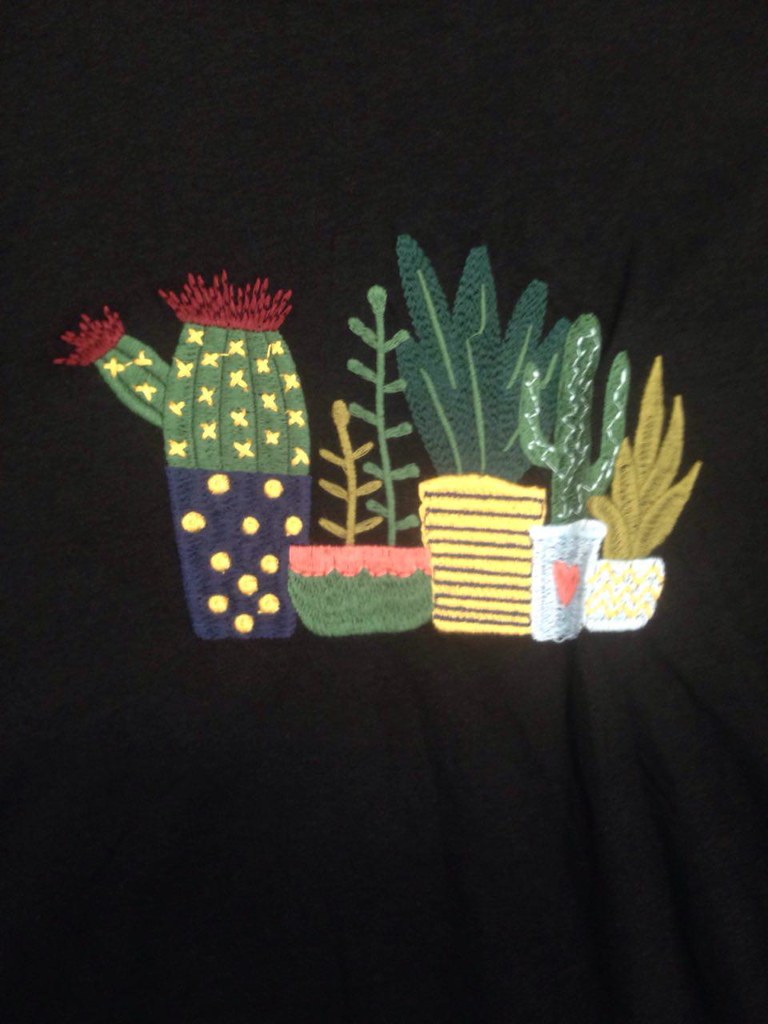Displayed against a solid black background is a fabric item adorned with intricate, sewn-on plant motifs. On the left, a striking large cactus with its distinctively broad shape catches the eye. To its right, two slender plants sprout from a pot, their thin leaves adding contrast to the broader foliage around them. Centered in the middle is a lush, green leafy plant that resembles a snake plant, characterized by its elongated leaves. Continuing to the right is a more traditional cactus, easily recognizable with its typical rounded form and spines. At the far right, there is another plant that appears to be either an aloe vera or another snake plant, contributing to the lush tapestry of greenery depicted on the cloth. The rich, black background enhances the vivid details and varied textures of the sewn-on plants, making them stand out strikingly.